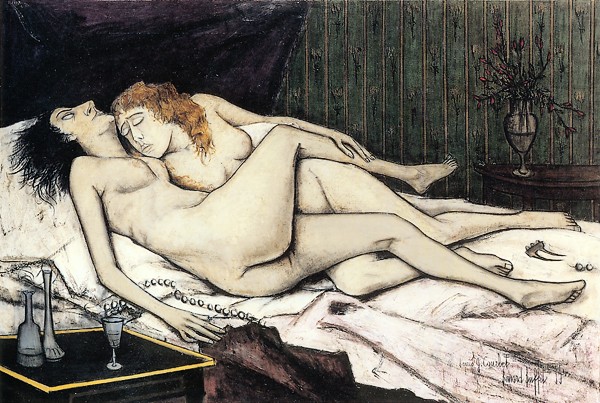A detailed painting depicts two women lying naked and intertwined on a white-sheeted bed. The woman lying on her back has dark black hair, while the woman resting on her chest has light brown, almost reddish-blonde hair. The scene, rich in contrast and detail, features a black night table outlined in yellow at the bottom left, adorned with a few gray objects, including some oddly shaped bottles and empty glasses. To the right, a dark gray vase holding black-outlined flowers adds a touch of elegance. The background presents a striking black wall that transitions into dark green wallpaper with faint flower patterns. In the foreground, closer to the viewer, lies a liquor glass and a bead of pearls nestled under the right arm of the nearer woman. This artwork, signed illegibly in the bottom right corner, captures an intimate and serene moment between the two women.